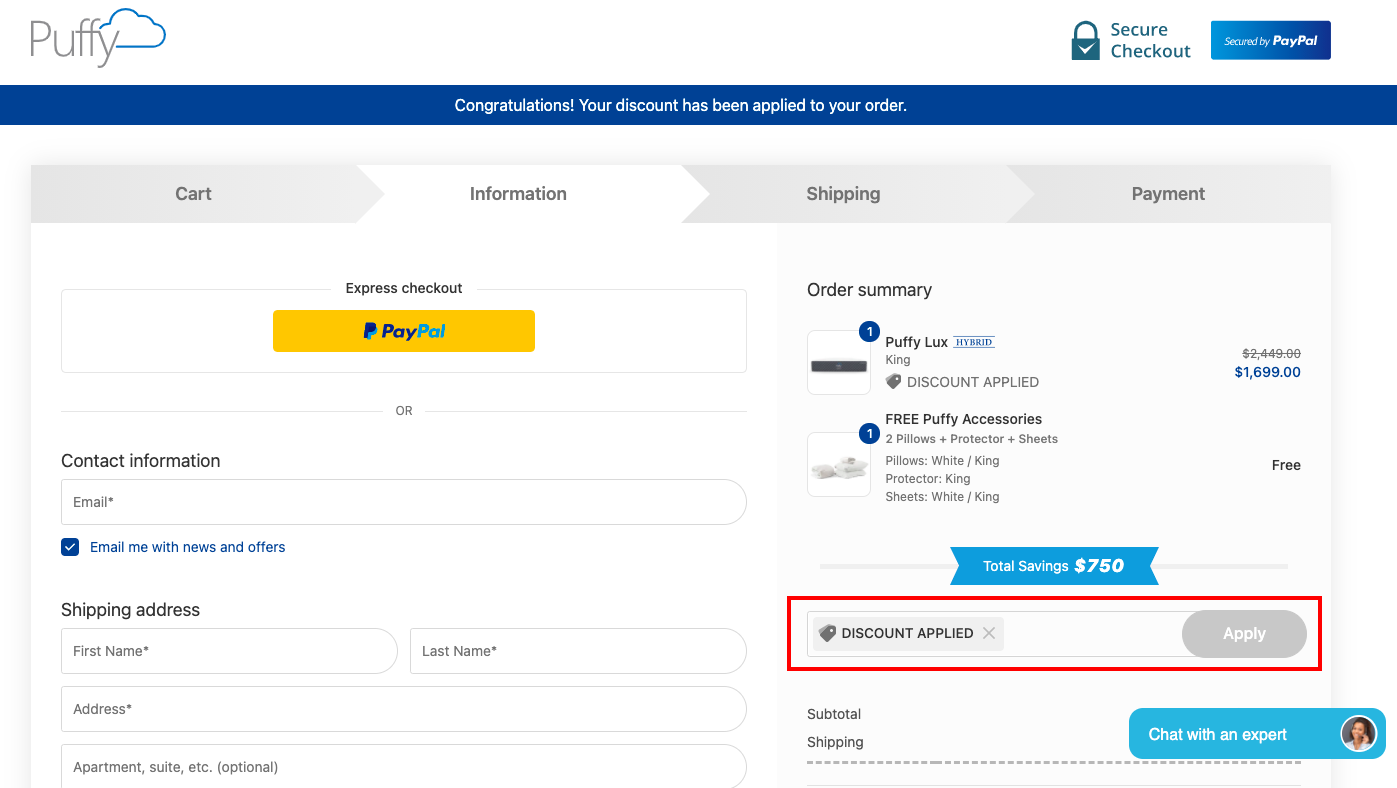The image displays a detailed section of the Puffy website's checkout page. On the left side, the Puffy logo, featuring the word "Puffy" accompanied by a cloud icon, is prominently showcased. To its right, text indicates a "Secured Checkout" process with a lock icon, followed by the guarantee "Secured by PayPal."

A blue banner below congratulates the shopper with the message, "Congratulations! Your discount has been applied to your order." Below this banner, navigation tabs labeled "Cart," "Information," "Shipping," and "Payment" are displayed, with the "Information" tab highlighted.

The section transitions into the "Express Checkout" option with PayPal, as well as a prompt for contact information, requesting an email address. There is also an option to subscribe for news and offers via email, crossed referenced in blue and linked.

Further down, the "Shipping Address" form requires filling out fields for the first name, last name, address, apartment (optional), and other relevant details. 

An order summary follows, listing items and savings. It specifies a "Puffy Luxe King" mattress with an original price of $2,449, now reduced to $1,699 after applying the discount. Additionally, it includes "Free Puffy Accessories" such as two king-sized white pillows, a protector, and white king-sized sheets, all marked as free. 

The total savings are highlighted as $750. The section concludes with a remark noting the discount application and finalization of the process.